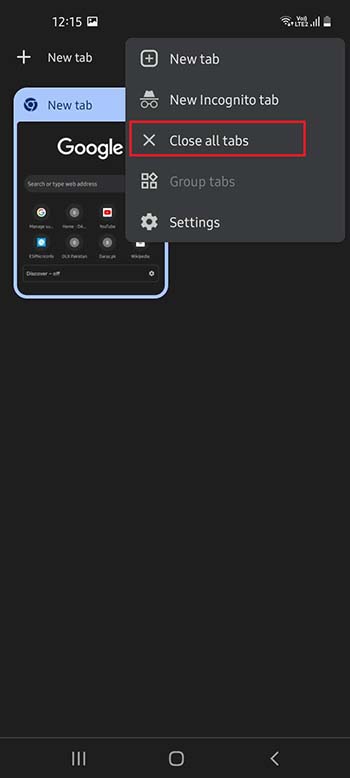The image features a predominantly black cell phone screen showcasing various interface elements. At the top left corner, the time "12:15" is displayed alongside a picture icon. To the right, status indicators for Wi-Fi signal, cellular signal bars, and a low battery level are visible. Just below, a toolbar includes a plus sign labeled "New Tab."

Central to the screen is a blue-outlined square labeled "New Tab" at the top, followed by the Google logo. In the upper right-hand corner of this Google section, a gray rectangular menu is partially visible. This menu contains options such as "New Tab," "New Incognito Tab," "Close All Tabs," "Group Tabs," and "Settings," with a red rectangle highlighting the "Close All Tabs" option, suggesting that this image is being used for educational purposes to demonstrate how to use this feature.

The remainder of the screen is largely black, with notable navigation icons at the bottom: three horizontal lines, a circle, and a left-pointing arrow—standard navigational elements on many smartphones. The image palette includes shades of black, blue, red, white, gray, and a hint of dark turquoise.